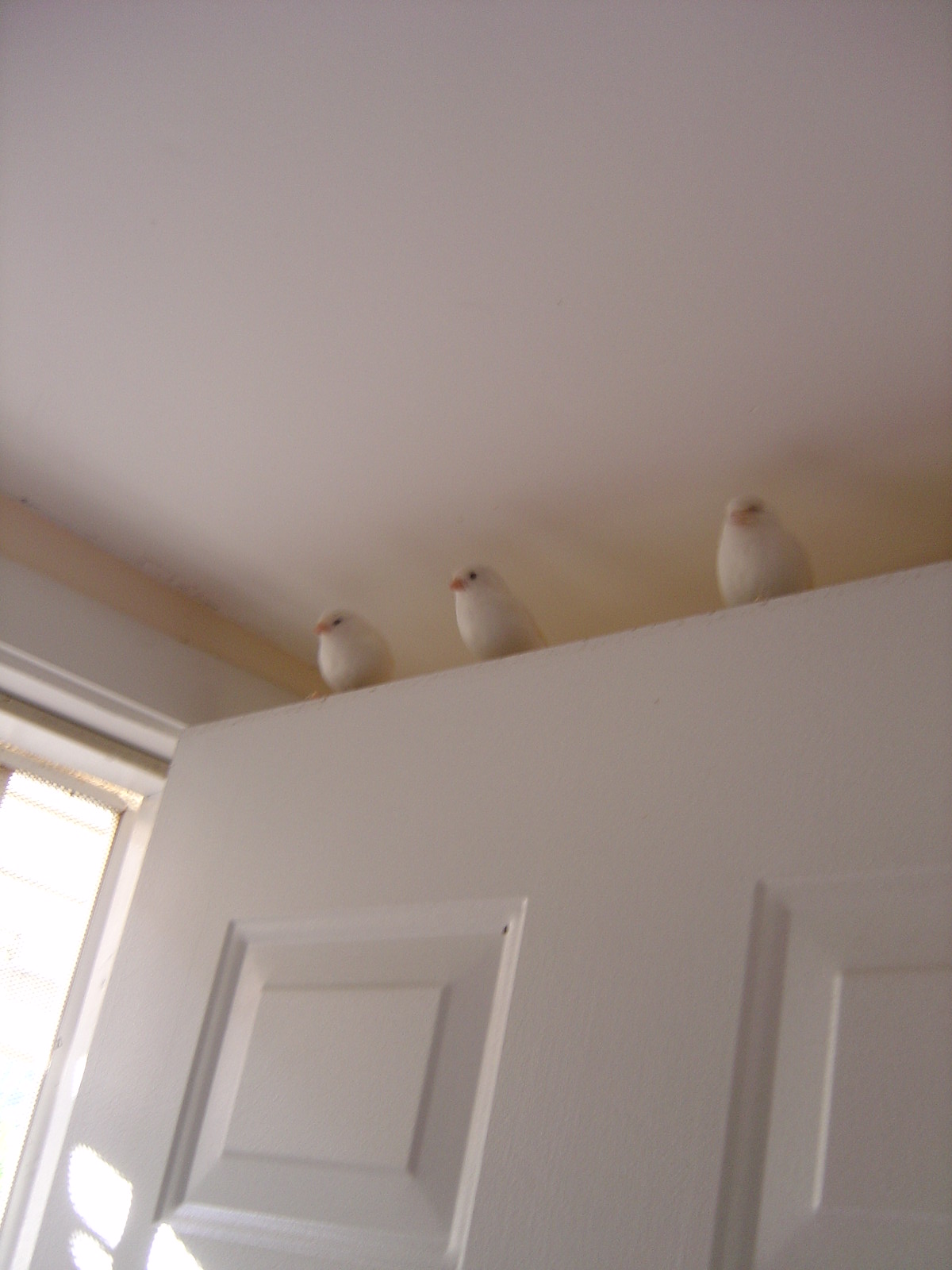The photograph shows a slightly blurry, portrait-oriented indoor scene centered on an open white wooden door with panels. The door, partially angled, appears narrower on the left side and wider on the right, cutting off about halfway through the image. Perched atop the door are three white birds, likely of the same species, characterized by their puffy appearance, small black or brown eyes, and orange or yellow beaks. These birds resemble doves or finches and stare straight ahead, seemingly brushing against the white ceiling due to their high perch. Bright sunlight streams in from the open doorway, creating a stark contrast with the shadows enveloping the door, the birds, and part of the room. The doorframe is also white, and the wall visible on the left side appears to be cream-colored.